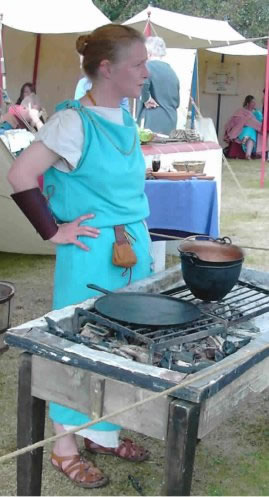In this image taken during the daytime, a woman with blonde hair, pale skin, and a blue dress or sweatshirt stands outdoors, possibly at a renaissance festival. Her outfit includes a leather bracer and pouches on her belt, and she has sandals on her feet. Her hair is pulled back, and she looks off to her right. Surrounding her are white canopies and tables as part of a makeshift outdoor marketplace or historical reenactment scene. In front of her, she stands by a wooden table, which holds a metal stove or griddle with a flat pizza-pan-like item and a black pot, suggesting she is cooking. The area is grassy, with several other people sitting or moving about in the background, emphasizing an active, communal atmosphere.